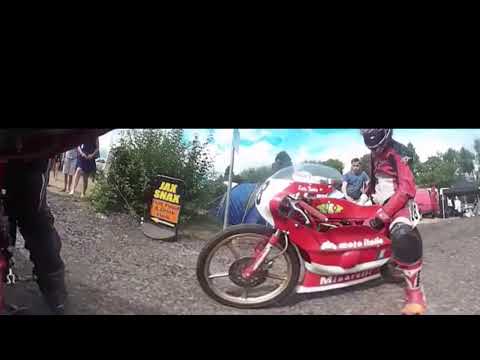In this vivid outdoor scene, a man wearing a red jacket, black knee pads, and a helmet sits astride a red motorcycle, which features a curved windshield. The motorcycle is parked on a gravel or dirt surface, surrounded by several people who appear to be hanging out or waiting in line. The setting suggests an event or gathering, possibly at a campground, evidenced by a red trailer, blue tent, and green bush in the background. To the motorcyclist's left, a yellow-lettered, black sign indicates directions to "Jack's Shacks" or "Jack's Snacks," with a white arrow pointing the way. The image is captured from an unusual angle, likely from a GoPro, causing a slight distortion and including more of the scene than what would typically be visible. The man behind the motorcyclist gazes at him, adding a dynamic human element to the otherwise static image.